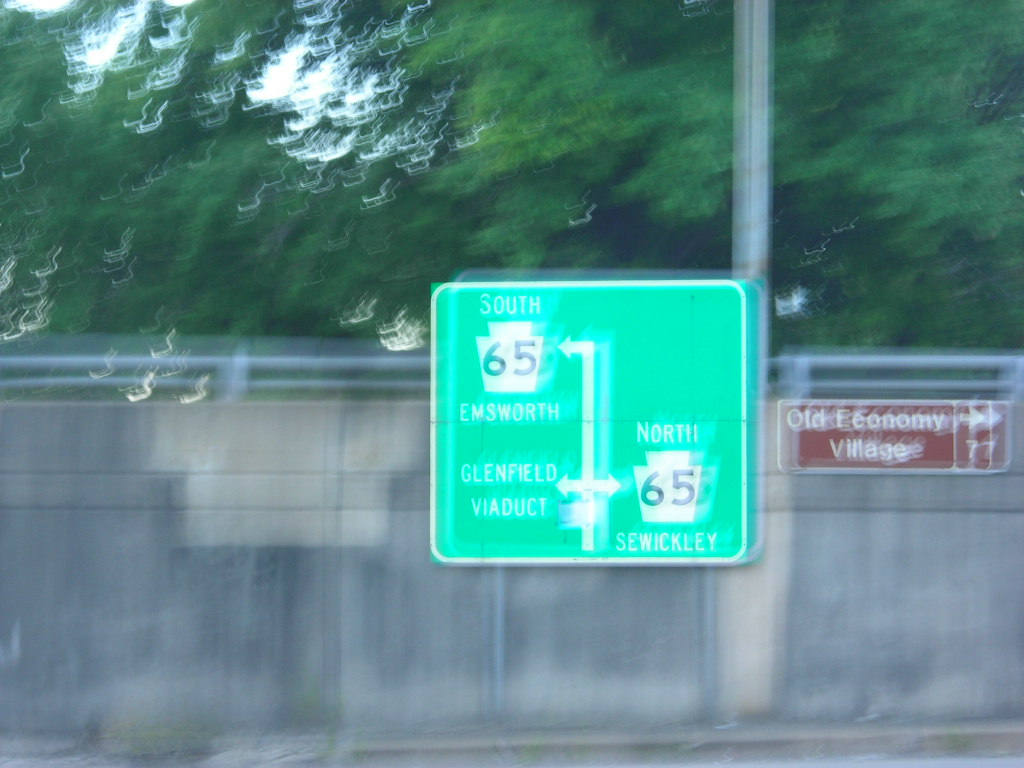The image depicts a highway bridge constructed from gray concrete or brick. Attached to the side of the bridge is a green, square highway sign with white text. The left side of the sign reads "South 65 Elmsworth," with an arrow pointing downward through the center. Adjacent to this is the text "Glensfield Viaduct," and to the right, "North 65 Sewickley." Additionally, there is a rust-colored, rectangular sign next to it, also with white text, indicating "Old Economy Village" and featuring a right-pointing arrow. Despite the photograph's blurriness and washed-out appearance, the background reveals a thick wall of green leaves and trees behind the bridge and signs, adding a natural contrast to the man-made structures.